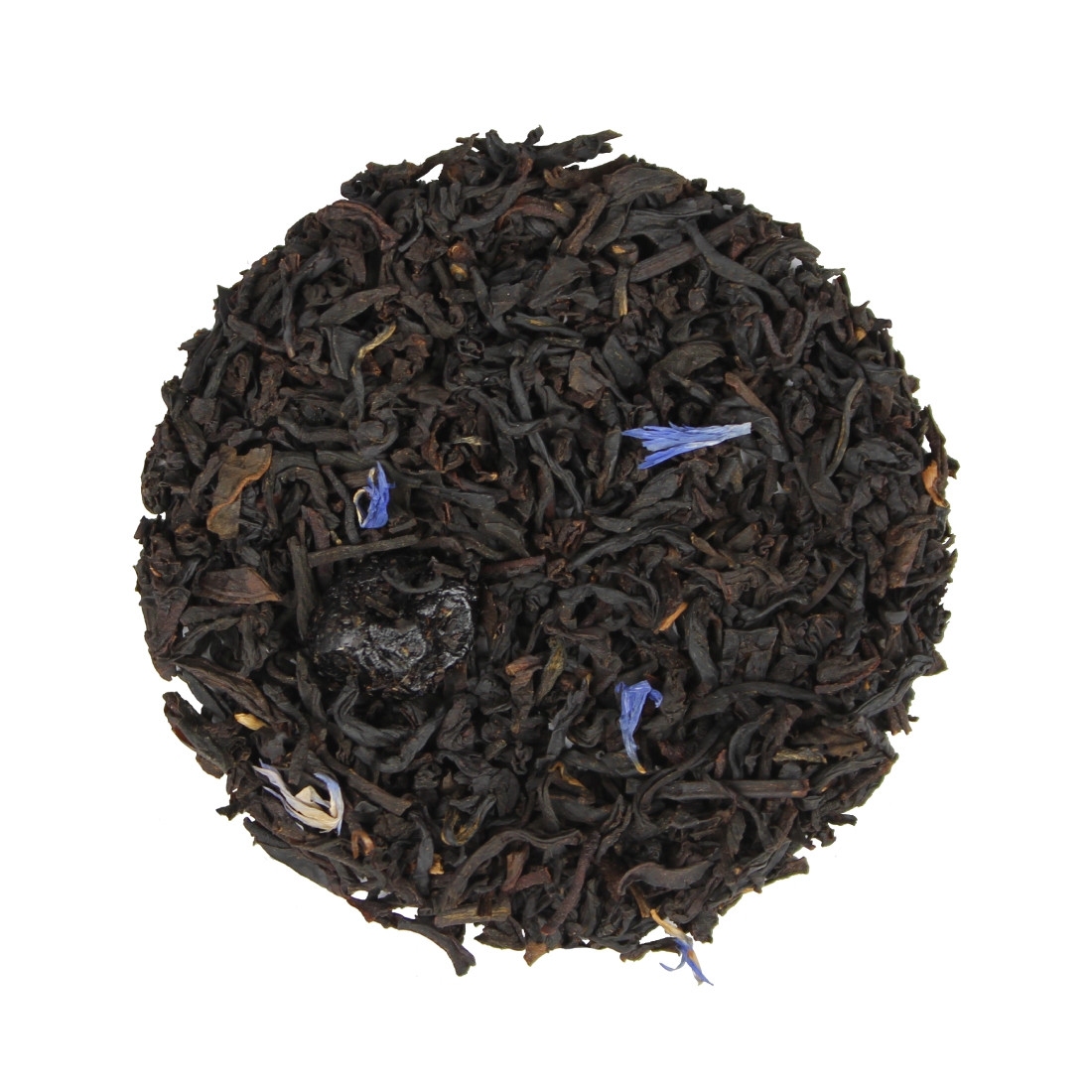The image depicts a meticulously arranged circular pile of decayed organic matter against a white background. The primary colors present include various shades of black and dark brown, resembling dried or possibly burnt plant material. Interspersed among this dark mass are remnants of more vibrant hues: light blue and purple flower petals are concentrated, forming a triangular pattern on the top, while a white petal is discernible on the lower left. Additionally, various leaves, seeds, and a grayish object resembling a stone are embedded within the pile, adding to the texture. This deliberate arrangement in a perfect circle suggests an intentional composition, perhaps to illustrate the contrast between life and decay from an overhead perspective.